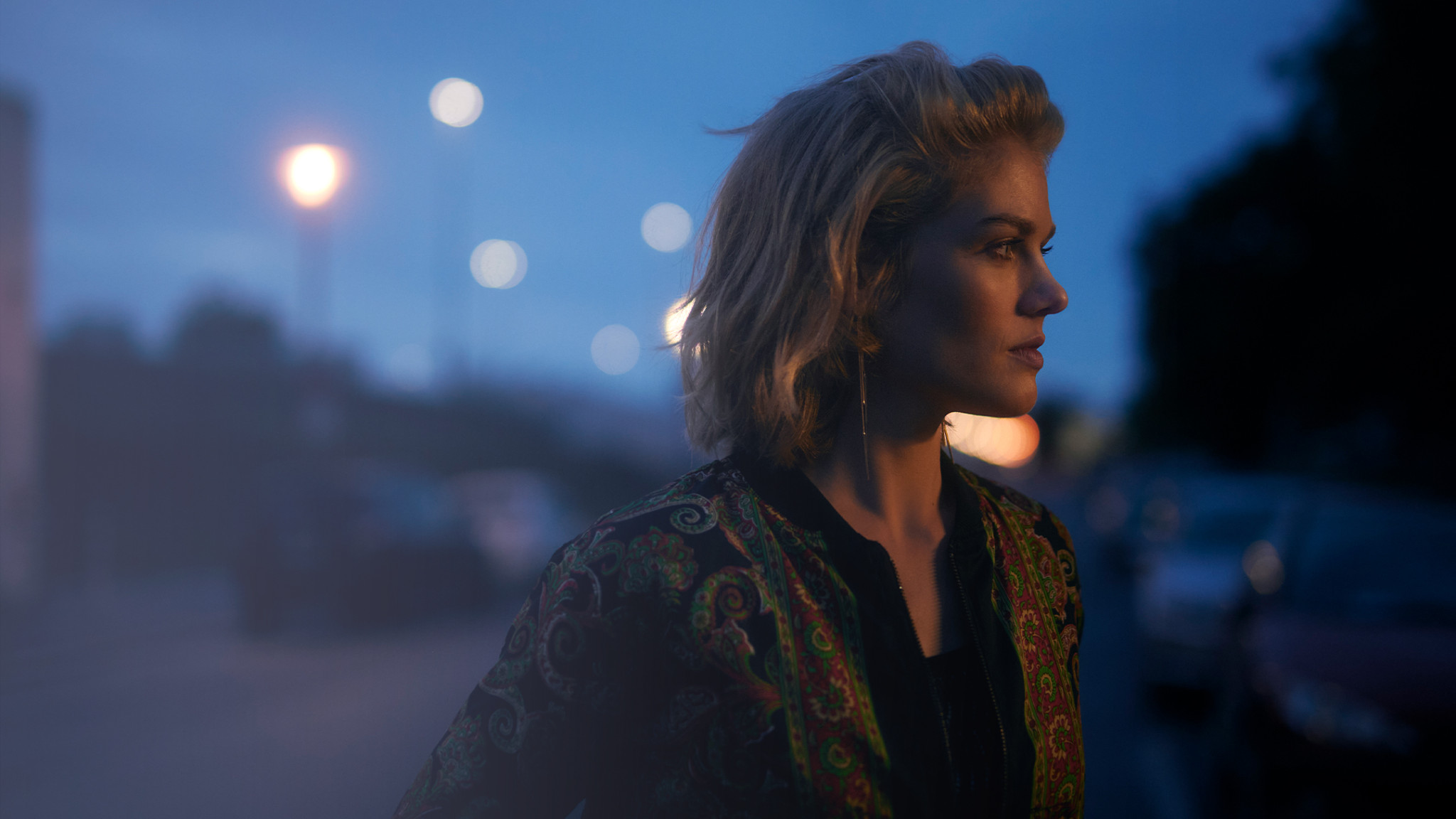The photo captures a young, Caucasian woman in a detailed side profile, standing outside at dusk on a blurry street. The scene is set in a landscape orientation, with the woman facing the right side of the image. Her shoulder-length blonde hair is pulled back, shimmering in the ambient golden light illuminating her face. She is dressed in a vibrant, paisley-patterned tunic jacket adorned with colors like navy, black, gold, green, and red, featuring a distinctive V-notch below the neck. Long, dangling earrings complement her attire. The backdrop, though out of focus, reveals a street lined with parked cars and illuminated by various streetlights and outdoor lighting poles. Her expression is pensive, and the composition emphasizes a sense of twilight realism.